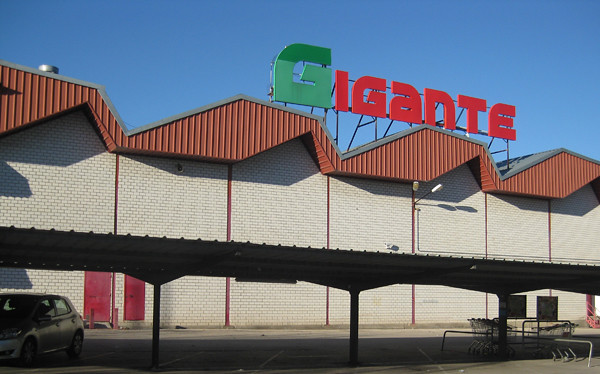In this clear, blue skies daytime photograph, we see an outdoor image of a retail supermarket named Gigante, spelled G-I-G-A-N-T-E, with the first G in green and the remaining letters in red. The building, centrally positioned in the image, is constructed of white brick with a prominent vertical red stripe that creates a paneled brick appearance. The roof above the building is distinctively orange-brown, swooping in undulating waves. Above the roofline, the store's name is displayed on a steel frame. In the foreground, a shaded carport area, partially cast in shadow, features a single vehicle parked on the left and several grocery carts to the right, underneath the cover. Additionally, the building has two red doors and is accented by spotlight fixtures extending from the wall.